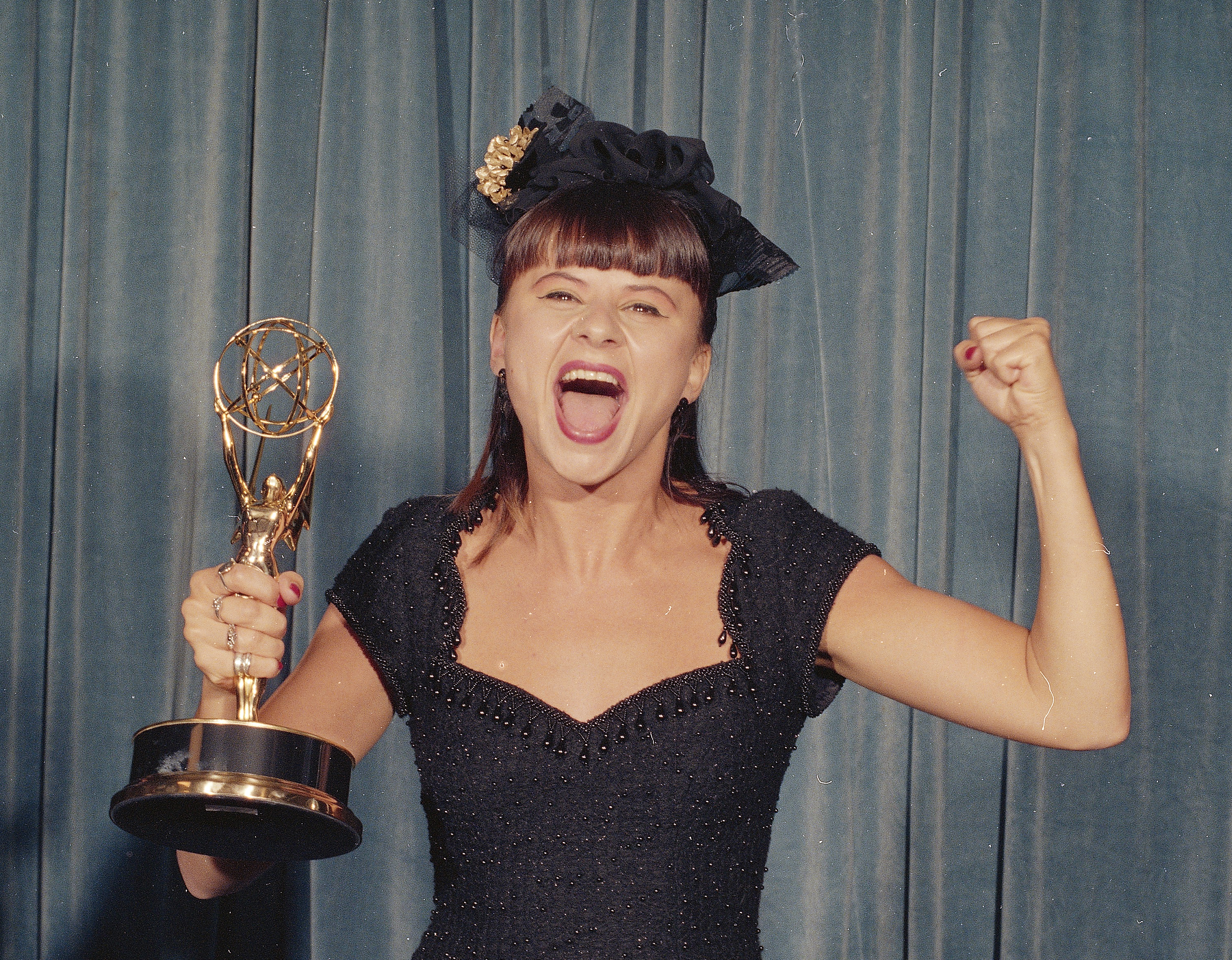The image features a young, jubilant woman, possibly in her 30s, who bears a resemblance to Rosie Perez. She is standing in front of a blue and gray curtain, capturing a moment of celebration at what appears to be an indoor awards ceremony. Dressed in an elegant black dress that is cut off at the shoulders, revealing her arms with red nail polish, she holds an Emmy Award—a gold statue of a woman holding a globe aloft—in her right hand. Her left hand is raised in a triumphant fist. She sports short reddish-brown hair with bangs, adorned by a black headdress accentuated with a gold clip, and her lips are painted a vivid red. The scene exudes joy as she looks towards the camera or audience, mouth open in a joyful shout, basking in the victory of her accolade.